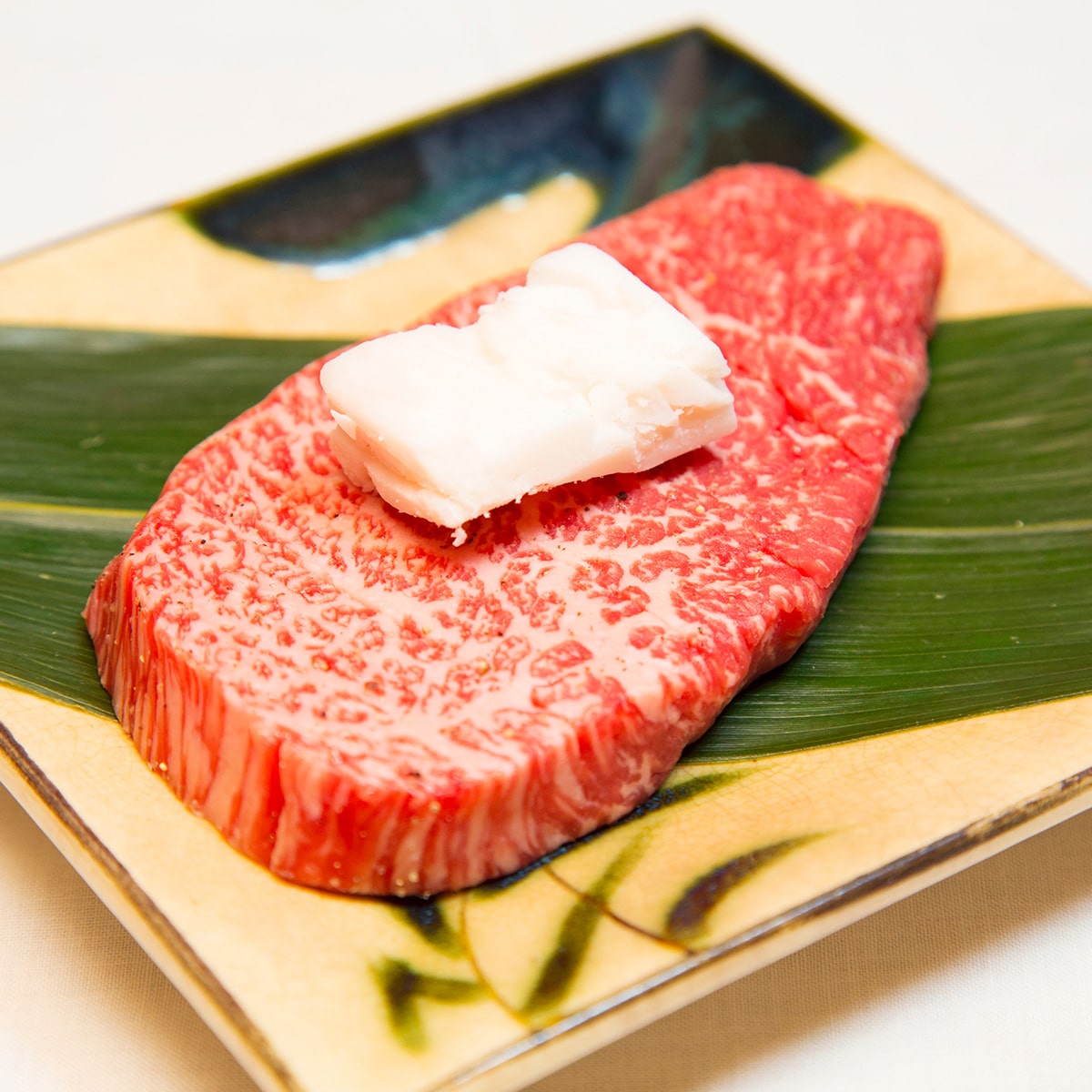This close-up image features a carefully arranged raw piece of meat, likely a highly marbled and fatty cut of wagyu beef, positioned on a square, beige-colored plate adorned with a leaf design. The plate is tilted about 45 degrees to the left, creating a dynamic presentation. A large green banana leaf stretches from the top left to the bottom right of the plate, while the beef, approximately an inch thick and richly marbled, is placed diagonally in the opposite direction. Atop the meat sits a substantial pat of white butter, enhancing its visual appeal. The entire setup, including the bamboo illustrations on the cutting board beneath, evokes an Asian culinary setting, suggesting that the meat is being showcased to highlight its quality before cooking. The absence of people in the image focuses all attention on the luxurious presentation of the meat itself.